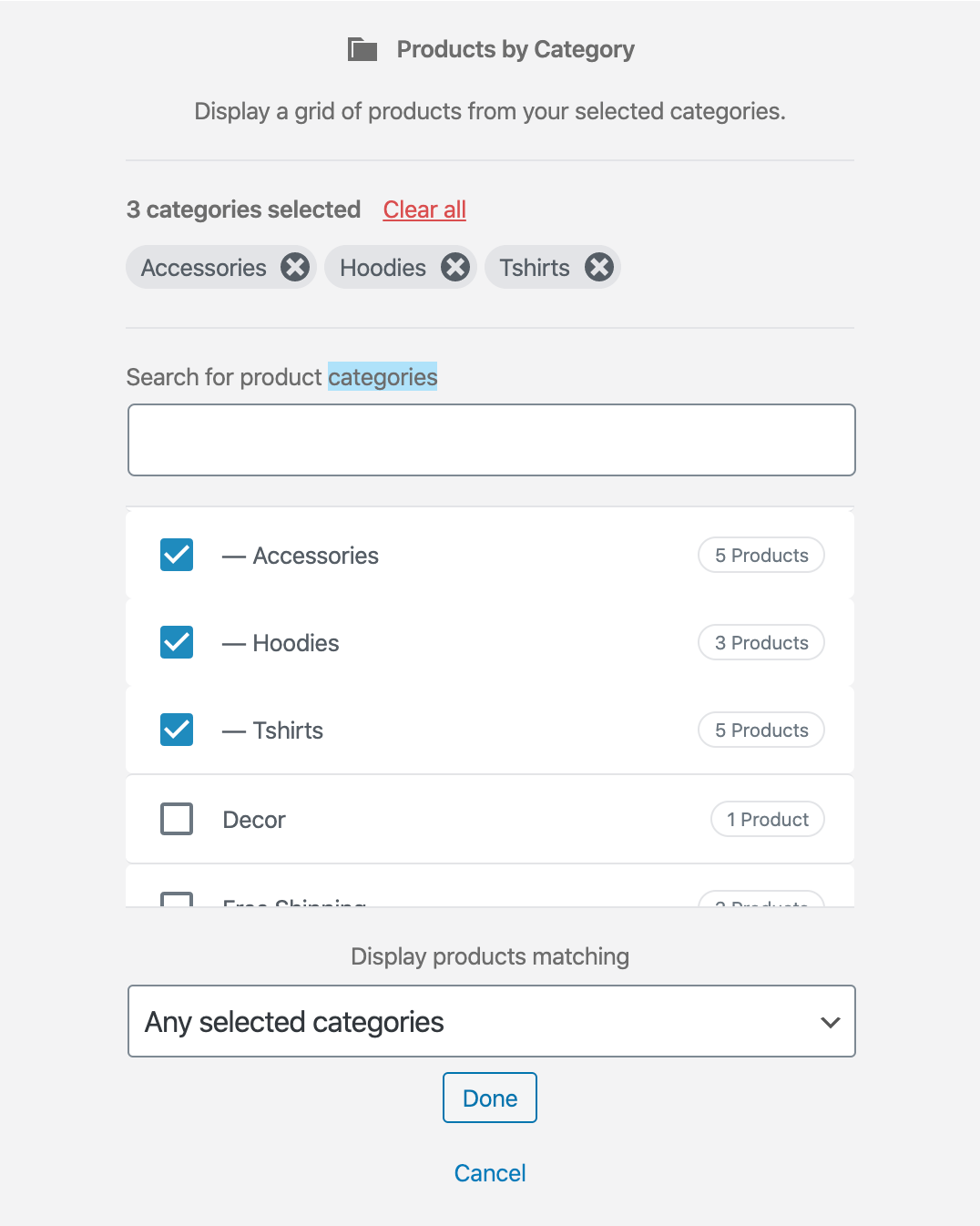The image features a layout with a gray border and various sections of text. At the top, a title reads "Products by Category," followed by an instructional subheading: "Display a grid of products from your selected categories." Beneath this, there's a descriptor indicating "Three categories selected," with an underlined, red "Clear All" option to the right-hand side.

Following that, three categories are displayed: "Accessories," "Hoodies," and "T-Shirts," each accompanied by an 'X' icon on the right for deselection. Below the categories, there's a search bar with the prompt "Search for product categories," where the word "Categories" is highlighted in blue.

The next section features a white rectangle listing the selected product categories: "Accessories," "Hoodies," and "T-Shirts." All have blue checked boxes to the left, and the respective product counts are indicated on the far right—five products for Accessories, three for Hoodies, and five for T-Shirts. Additionally, there's an unchecked "Decor" category at the bottom, indicating it has one product.

Further down, in the gray section again, there is a label reading "Display products matching," accompanied by a drop-down menu set to "Any selected categories." Below is a small rectangle with the word "Done" in blue, and underneath it, the word "Cancel" is also in blue.